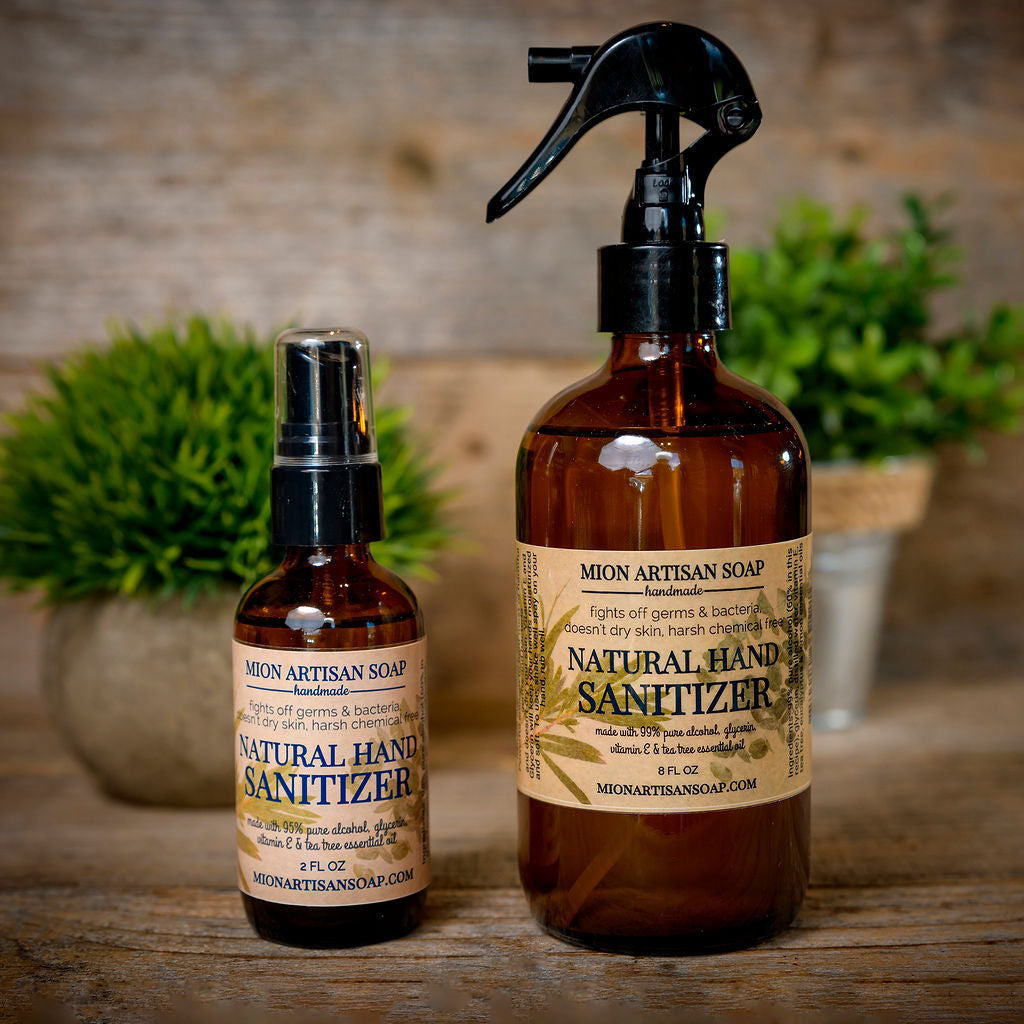This image showcases two bottles of natural hand sanitizer from Neon Artisan Soap. The bottles, one small (2 fl oz) and one large (8 fl oz), are made of brown glass with black plastic sprayers. The labels on both bottles emphasize their handcrafted nature and benefits, highlighting that they fight off germs and bacteria, do not dry the skin, and are free from harsh chemicals. The formula includes 99% pure alcohol, glycerin, vitamin E, and tea tree essential oil. The website neonartisansoap.com is printed at the bottom of the labels. The smaller bottle features a standard spray top encased in clear plastic, while the larger bottle has a more robust, handle-style sprayer. The bottles are set on a light wooden table, and in the blurred background, there are two potted plants—one in a large, stone-like circular pot and the other in a slender vase. Behind the plants, there appears to be a wall with a ledge, adding depth to the scene.